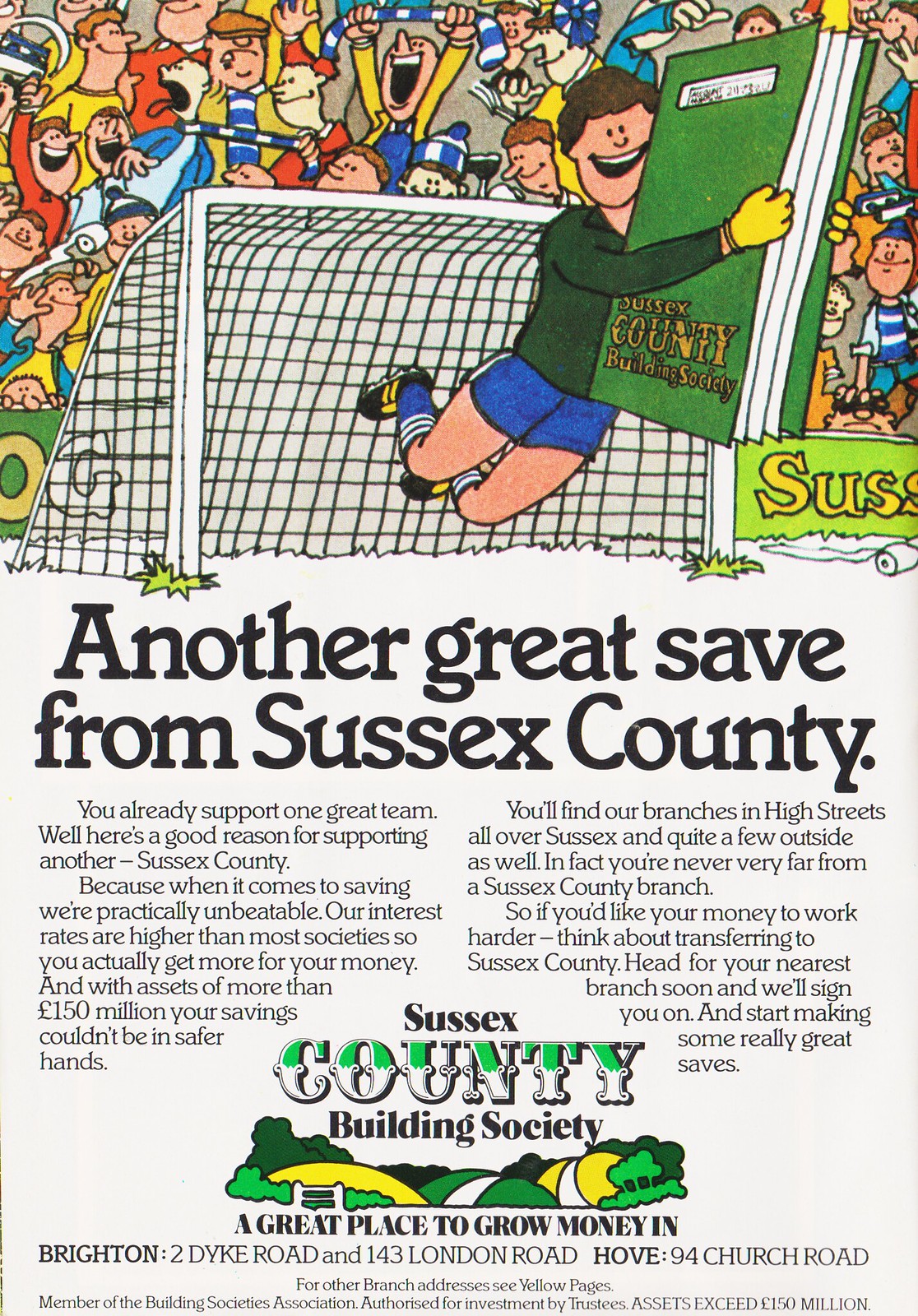This is a detailed cartoon image showing a soccer player making a dynamic save in front of a white goalpost. The player, dressed in green with blue shorts and socks, has leaped up to catch a large green book labeled "Sussex County Building Society" in yellow text at the bottom. Behind him, cartoon fans cheer enthusiastically.

Below the scene, the title "Another Great Save from Sussex County" is prominently displayed in black text. 

Underneath the title, two paragraphs detail an advertisement for Sussex County Building Society. The left paragraph encourages readers to support Sussex County, emphasizing the tagline, "When it comes to saving, we’re practically unbeatable." It highlights their higher interest rates and mentions their impressive assets of over 150 million, ensuring the safety of savings. 

The second paragraph elaborates on the accessibility of their branches, scattered across Sussex and beyond, and promotes transferring savings for better returns, inviting potential customers to their nearest branch. 

At the bottom, in white and green letters, the text reads "Sussex County Building Society – A great place to grow money in," followed by addresses at 2 Dyke Road, 143 London Road, and 94 Church Road. The backdrop features scenic country land, reinforcing the association with community and growth.